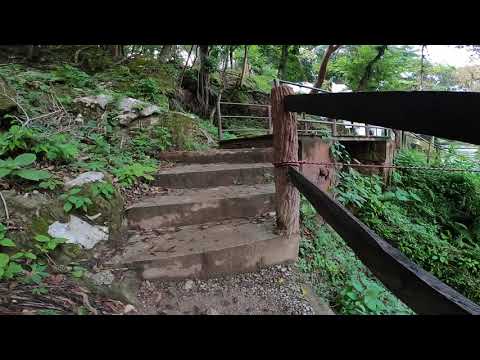The photograph depicts a bright daytime scene set on a rocky hillside that transitions into a lush, jungle-like area, potentially near an urban environment. A pathway with cement and stone steps ascends through this natural landscape, bordered by a wooden fence railing. The rocky terrain around the steps is alive with a variety of weeds, shrubs, and small plants boasting large green leaves, all of which add to the dense, jungle-like ambiance. On the right side of the stairs, thick foliage dominates the area, while the left side is adorned with smaller plants and pebbles. Further up the steps, a wooden or possibly metal bridge extends into the distance, blending into the forested backdrop. In the far right distance, amidst the thick layer of trees, the silhouettes of numerous buildings can be faintly seen, indicating a nearby cityscape. The image is distinguished by black horizontal bars across its top and bottom, framing the vibrant outdoor scene.